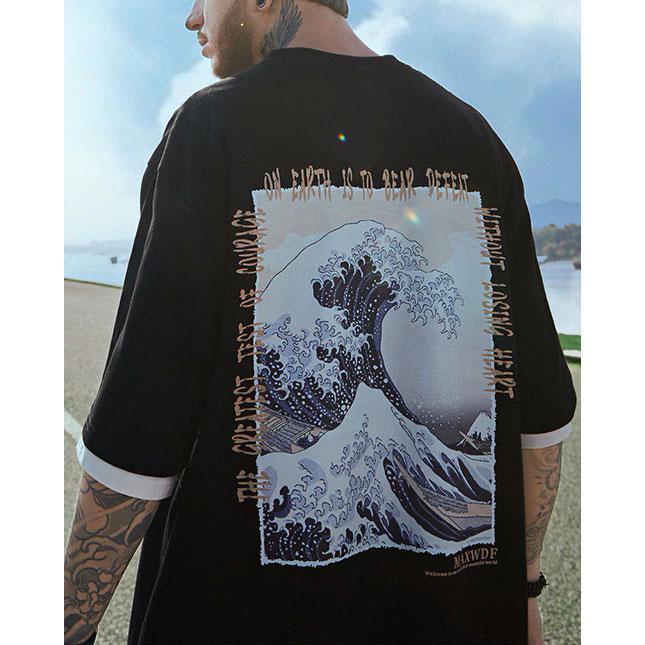The image depicts a man viewed from the back, with only the bottom part of his earlobe and a light mid-brown beard visible as he faces away from the camera. His slightly visible profile reveals a black earplug in his left ear, and an elaborate green feather-like wing tattoo extends from his neck toward his hairline. Both of his arms are partially cut off in the frame, adorned with intricate dark green and black swirl tattoos, and he wears a black strap, likely a watch, on his partially obscured right hand.

He is dressed in a black T-shirt with white bands just below the elbows. The back of the T-shirt prominently features a portrait-style image of white and dark navy blue crashing waves, surrounded by difficult-to-read orangey-beige text. The clearer portion of the text at the top reads, "On earth is to bear defeat without losing heart," while other text along the sides and bottom, such as "maxwdf," remains somewhat illegible due to the low quality and wavy fabric.

In the background, the sky is a vibrant blue with scattered clouds, and a mixture of gravel or beach-like surface covers the lower part of the scene. The overall setting suggests the man is standing in an open, outdoor area, possibly near a beach or a similar location.